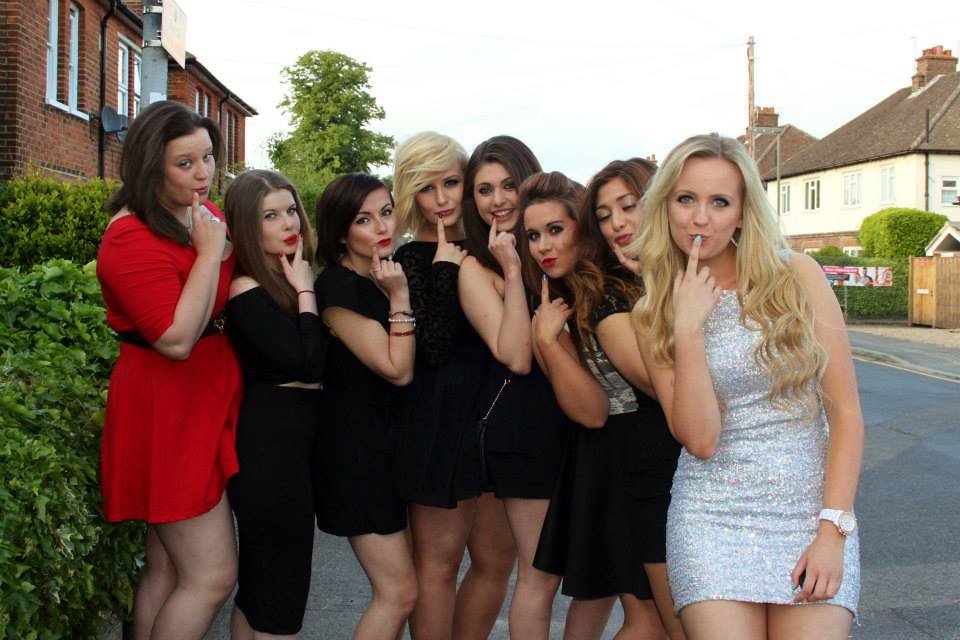In this daytime photograph, eight women aged approximately 20 to 30 are standing together, seemingly ready for a party, prom, or dance. They are posing coyly for the camera, each with a finger up to their mouth. The women are standing on a sidewalk in a neighborhood with brick buildings and homes behind them, flanked by green bushes. Six of them are wearing black dresses, the woman on the far left stands out in a red dress, and the woman on the far right shines in a sparkly white and silver dress. They are all white with varied hair colors, including six brunettes and two blondes.